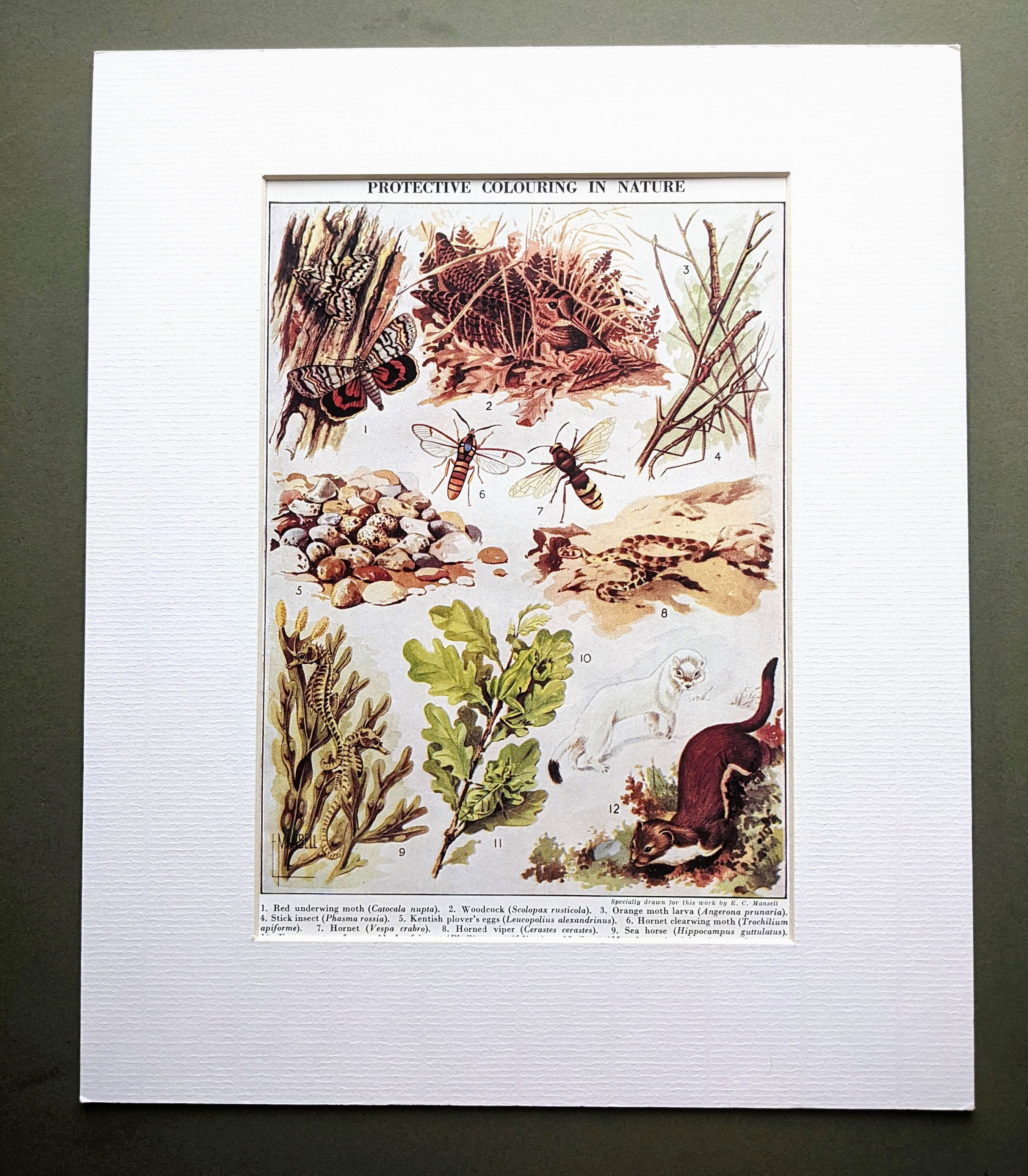The image is a rectangular illustration roughly six inches high and five inches wide, encased in a matte gray background. A thick white cardstock border with subtle horizontal ridges surrounds the illustration. At the top, black text on a white background reads "Protective Coloring in Nature." The detailed, old-textbook-style drawings feature various examples of camouflage in nature, including animals, insects, and plants. Each illustration is numbered and labeled, though some lower numbers are partially obscured by the frame. Specific examples include a red underwing moth, woodcock, orange moth larva, stick insect, Kentish plover's eggs, hornet clear wing moth, hornet, horned viper, and seahorse. Additional illustrations, possibly of a frog, white ferret, and brown ferret or otter, are also visible. The entire collection of illustrations is surrounded by a thin black border within the frame.